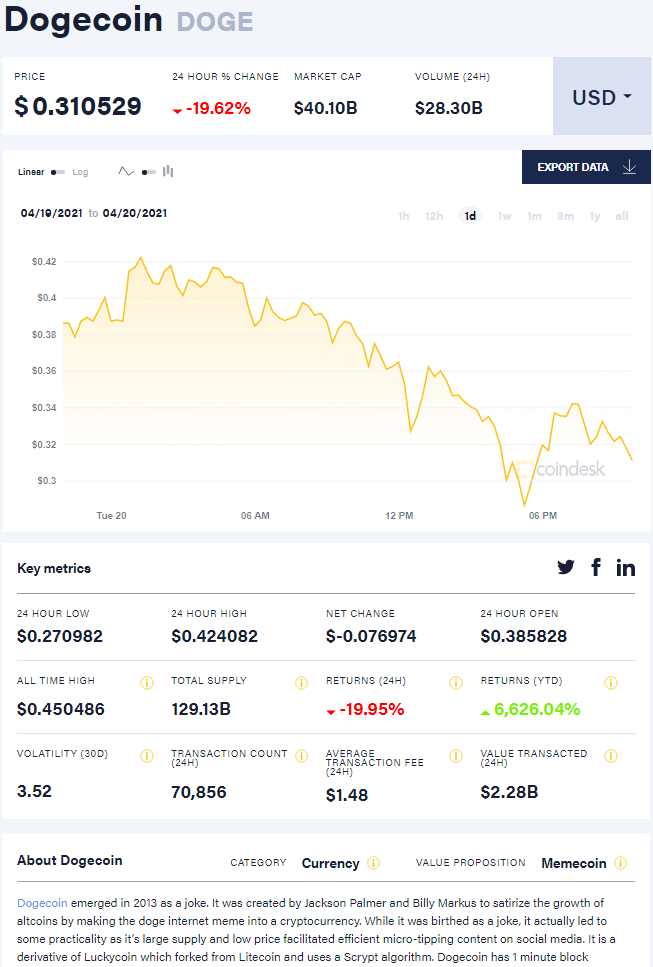The image showcases a comprehensive interface for tracking Dogecoin (DOGE) metrics, likely displayed on a financial website or app. The background features a gradient of gray tones with a black banner at the top. Within the banner, the "Dogecoin" name is displayed in a bold, modern font, accompanied by a darker gray Dogecoin symbol.

Beneath this banner, there's a prominent white background section divided into four columns:

1. **Price:** Displays "Price: $0.310529."
2. **24-Hour Percent Change:** Indicates a change of "-19.62%" with a downward arrow.
3. **Market Cap:** Lists "Market Cap: $40.10 Billion."
4. **Volume in 24 Hours:** Shows "Volume in 24 Hours: $28.38 Billion."

To the far right of these columns is a dropdown menu set to "USD" (United States Dollar), allowing users to switch currencies if needed.

Below these metrics is a chart displaying a downward-trending line graph, representing DOGE's price change over the last several hours. On the top right corner of the chart, users can find an "Export Data" button. On the left side, there are buttons for logging in and toggling between different types of graphs (line or bar).

The interface also includes a table with key metrics located beneath the graph, giving users further detailed information about Dogecoin's performance.